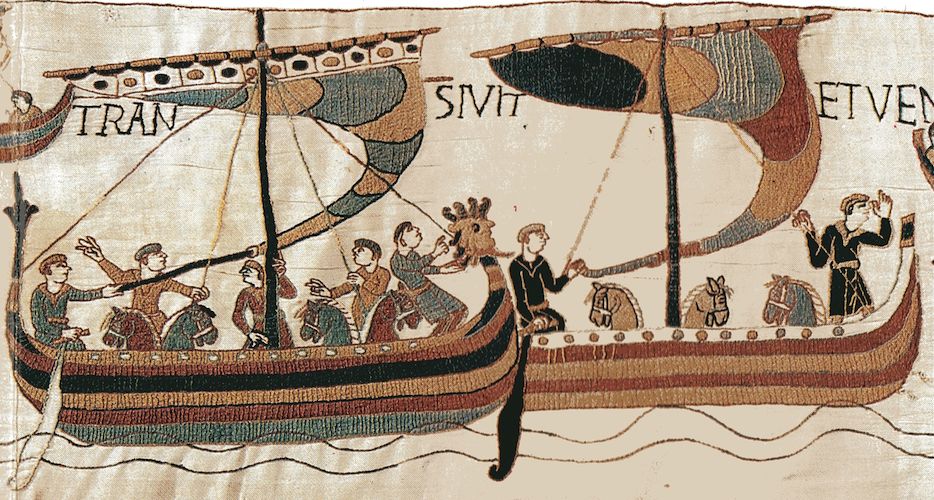This image depicts an ancient scene on a canvas sheet, likely made of animal hide, featuring two ornate boats. Each boat, shaped like traditional canoes, is adorned with colorful stripes in shades of tan, brown, green, and light blue. The boat on the left carries about six people and four horses, while the boat on the right has two people and three horses, with the horses' heads prominently visible. Both boats possess sails that are intriguingly shaped like large megaphones or horns. The background is a light tan color, resembling an old piece of fabric with intricate stitch designs. Near the bottom, two thin brown lines represent water waves, enhancing the scene's depiction of a voyage. Above the boats, an inscription reads "TRAN SIVIT ETVEN," potentially in Latin, suggesting an ancient cultural origin.